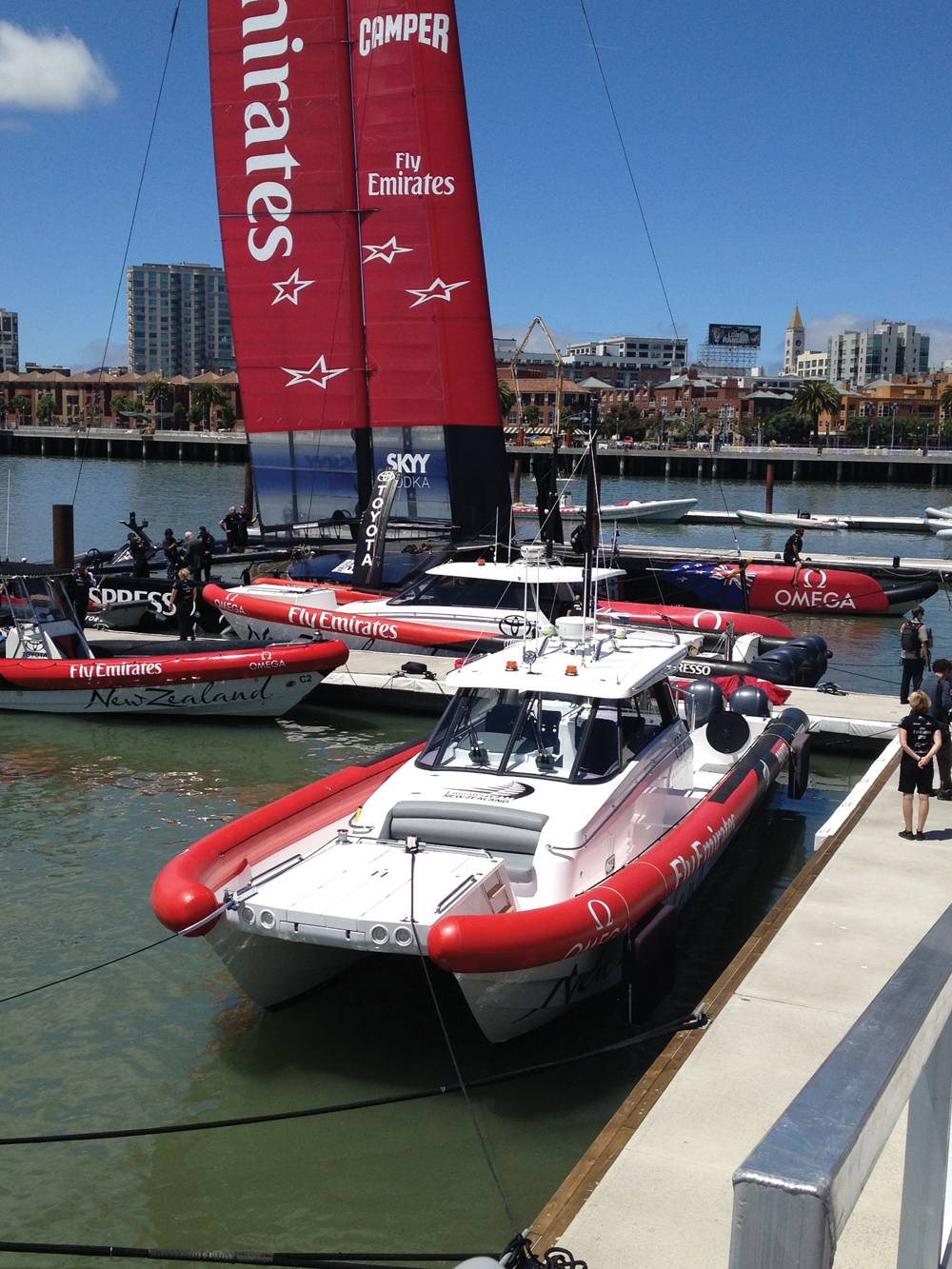In this photograph, the foreground features a prominent white dock that serves as the focal point. Moored at the dock is a small, white catamaran approximately 25 feet in length. This catamaran is adorned with red bumper-like fenders and bears the inscription "Fly Emirates" on its side. Surrounding the main catamaran are three or four other boats, similarly colored in red and white, and also displaying the "Fly Emirates" branding. One of these boats is distinctly marked with “New Zealand.” A strikingly tall structure, possibly a windjammer sail or a pier marker, dominates the scene with its red and white design and the "Fly Emirates" logo. In the distance, a city skyline offers a contrasting backdrop to the busy dock area.